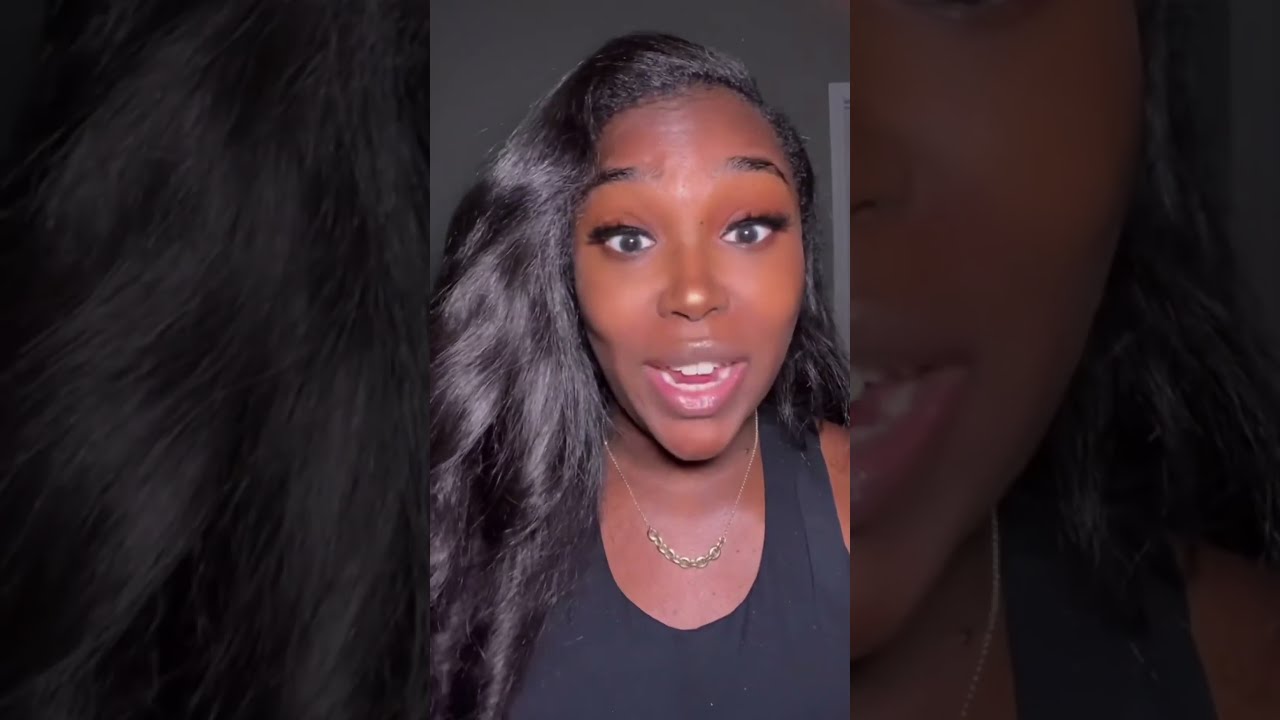The image is a vertical, cellphone-style picture divided into three equal rectangular segments. The central segment features a young African-American woman with a glossy, oval face. She has long, straightened black hair, parted on the side and swept into large spiral curls over her right shoulder. Her expression, captured mid-conversation, is one of slight surprise, with raised eyebrows and almond-shaped eyes framed by thick false eyelashes. This highlights her natural expression rather than actual surprise, as the whites of her eyes are visible only left and right of the irises. She wears a black sleeveless tank top and a delicate gold necklace, possibly with some small embellishments or lettering that aren't clearly visible due to distance. Her lips are glossed, adding to her polished appearance.

The left and right segments of the image are blurred, darkened, and zoomed-in portions of the main central image, serving as its backdrop. The left side prominently features an up-close shot of her shiny black hair, while the right side shows an enlarged view of her lower face. In the background, a gray ceiling is visible, providing a subtle context to the setting.